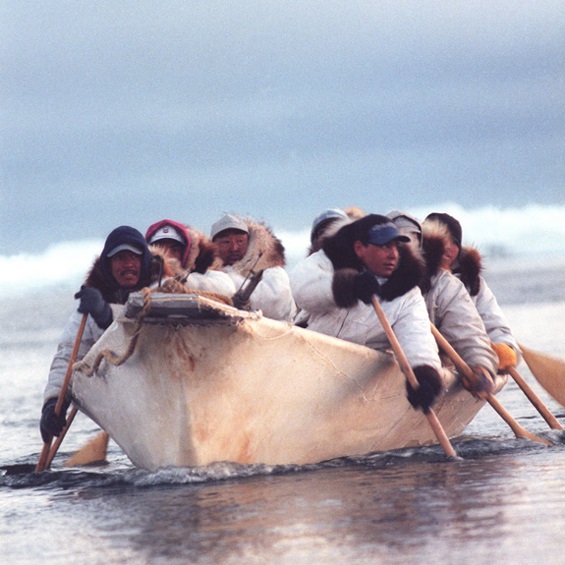The photograph captures a group of approximately eight men rowing a white canoe-like boat in icy ocean waters, likely in an Arctic setting. The boat, traversing towards the camera, features three men on the right side and three men on the left, with possibly one person positioned at the back. All the men are uniformly dressed in heavy white puffer jackets with brown fur collars, gray fur gloves, and gray baseball caps, suitable for the cold climate. One individual on the left side is distinguishable by a black-white jacket and a gray cap, while another on the left features a jacket with a red-bordered collar. The scene also includes another canoe partially visible in the background. The clear, slightly overcast blue sky and distant white caps further enhance the serene yet frigid atmosphere of the image.